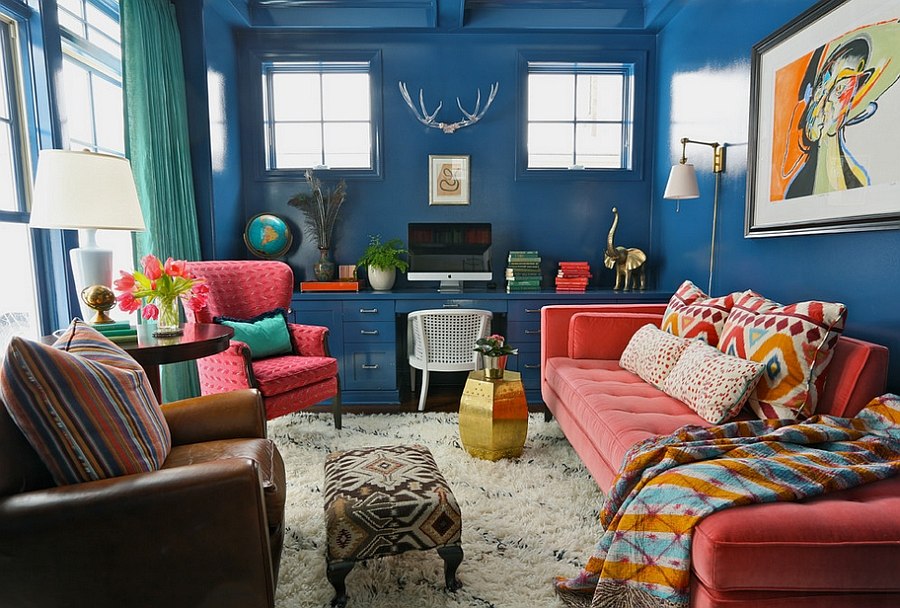This is an image of a vibrant and colorful living space, which seems to function both as a living room and an office, likely within an apartment. The room features large, floor-to-ceiling windows on the left wall, allowing ample natural light to pour in. The remaining walls are painted a robin's egg blue, complementing the room’s bright and lively atmosphere.

Towards the far end of the room, there is a blue desk positioned centrally. On the desk, a Mac computer is flanked by stacks of books and an elephant statue on the left, with various small items such as a globe and a lamp enhancing the decor. Above the computer, there are two mirrors and a pair of hunting trophy horns mounted on the wall, adding unique touches to the space.

The seating area includes a mix of colorful furniture: on the right, an elongated orange sofa with vividly patterned pillows in shades of red, beige, purple, orange, and blue; on the left, a brown sofa and a red sofa complement each other, while individual leather chairs are placed near the windows. The room is decorated with various artworks and pictures on the walls, enhancing the overall aesthetic with a broad spectrum of colors, including light reddish-pink, mint green, ocean blue, and yellow. Each element of the room, from the furniture arrangement to the decorative accents, contributes to the dynamic and eclectic feel of this multifunctional living and office space.